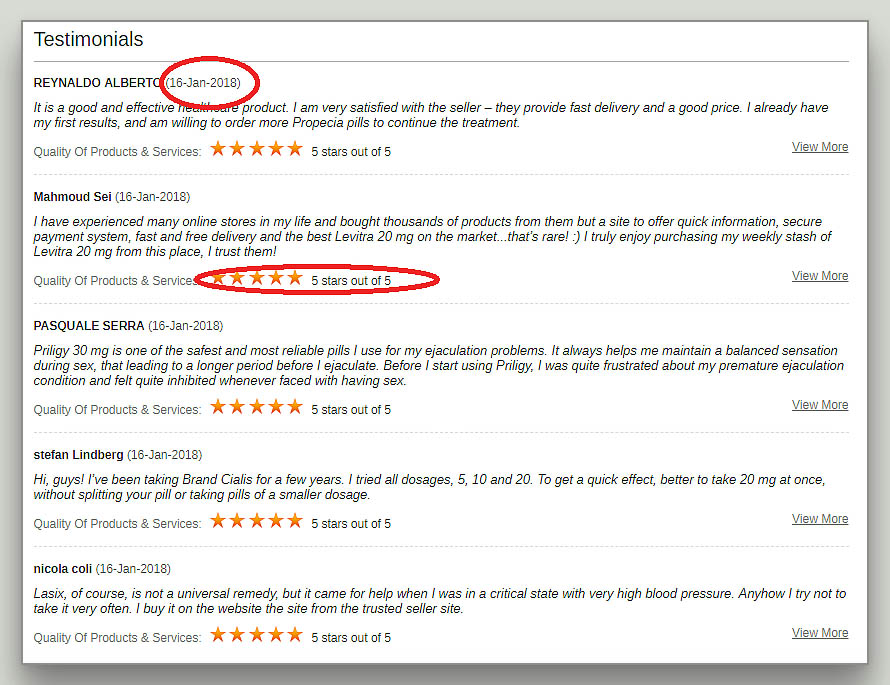This screenshot showcases a series of testimonials, each rated five out of five stars, for an online pharmacy. In the upper left corner, the word "Testimonials" is prominently displayed. A date, January 16, 2018, is circled in red, emphasizing the recency of the feedback.

The first testimonial is by Reynaldo Alberto, who expresses high satisfaction with the product and service. His testimonial reads: "This is a good, effective product. I am very satisfied with the seller—they provide fast delivery and a good price. I already have my first results and am willing to order more Propecia pills to continue the treatment." He awarded the seller a perfect five-star rating.

Following Reynaldo's review, another testimonial is highlighted, also circled around the five-star area. This praise comes from Mamoud Sey on the same date, January 16, 2018.

Subsequent testimonials include praise from Pasquale Sara, Stefan Limburg, and Nicola Koli, all dated January 16, 2018, consistent with the other reviews. Each of these reviewers assigned a five-star rating to their experience with the pharmacy.

The reviews mention various medications such as Priligy 30 mg, Levitra 20 mg, and Lasix, indicating the pharmacy's diverse product offerings. This compilation of testimonials emphasizes the high level of customer satisfaction and efficient service provided by the online pharmacy.